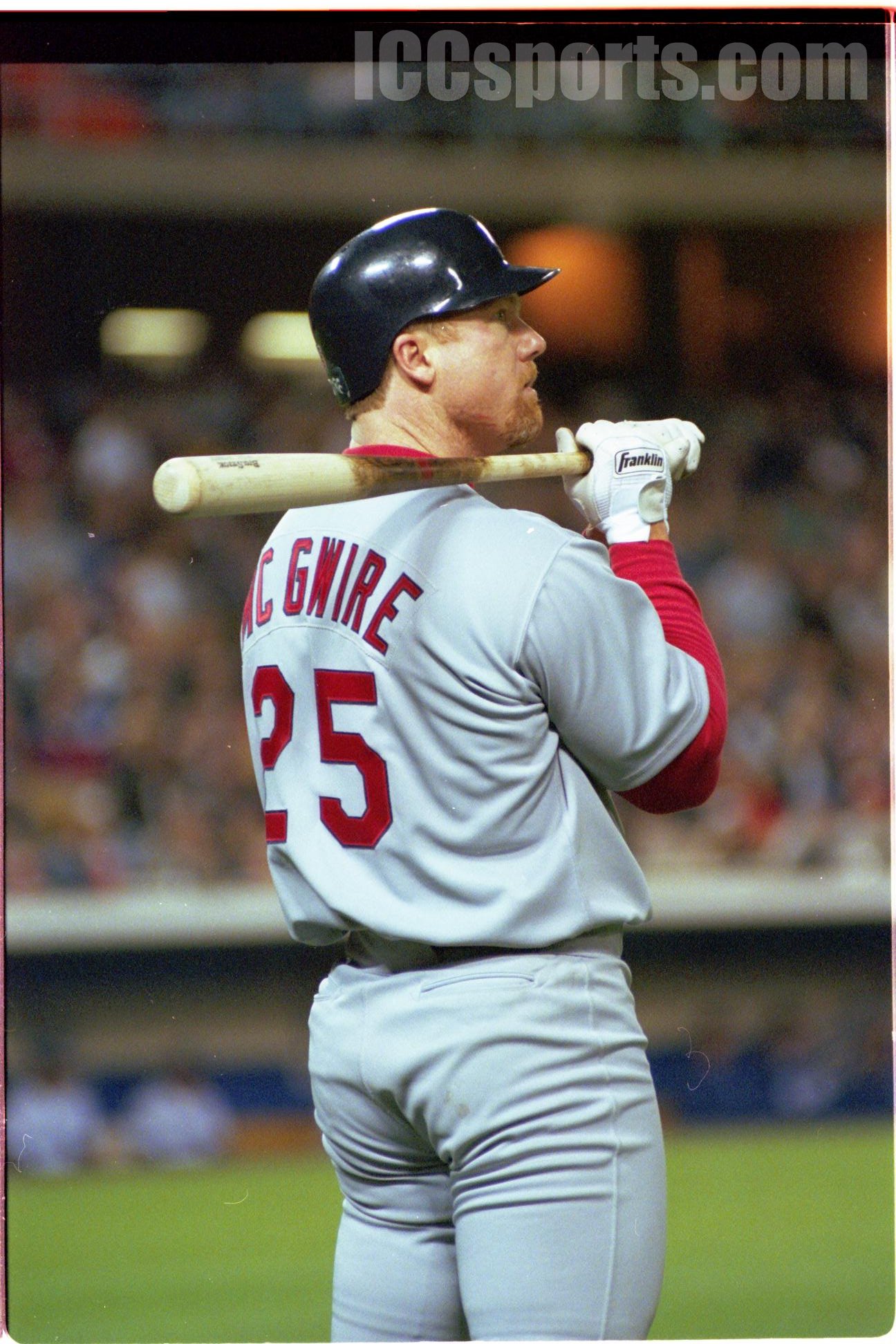This tall, rectangular photograph captures a Major League Baseball player from his thighs up, facing right with his body angled diagonally. The player, identified as Mark McGuire, renowned former home run champion who played for the St. Louis Cardinals, is seen intently watching the play, presumably from the on-deck circle. He sports a dark helmet, red hair, and a red beard. His uniform is gray with red lettering, featuring the number 25 prominently on the back with "McGuire" displayed above it in a curve. Underneath his uniform, he wears long red sleeves, complemented by tight, gray pants that bunch slightly at the back. McGuire grips a light brown wooden bat, which rests over his left shoulder, marked with noticeable pine tar. He also wears white batting gloves inscribed with "Franklin" in black font. The background reveals the stands and dugout with a hint of green grass at the stadium, accentuating the scene with an ambient atmosphere of an awaiting baseball moment.